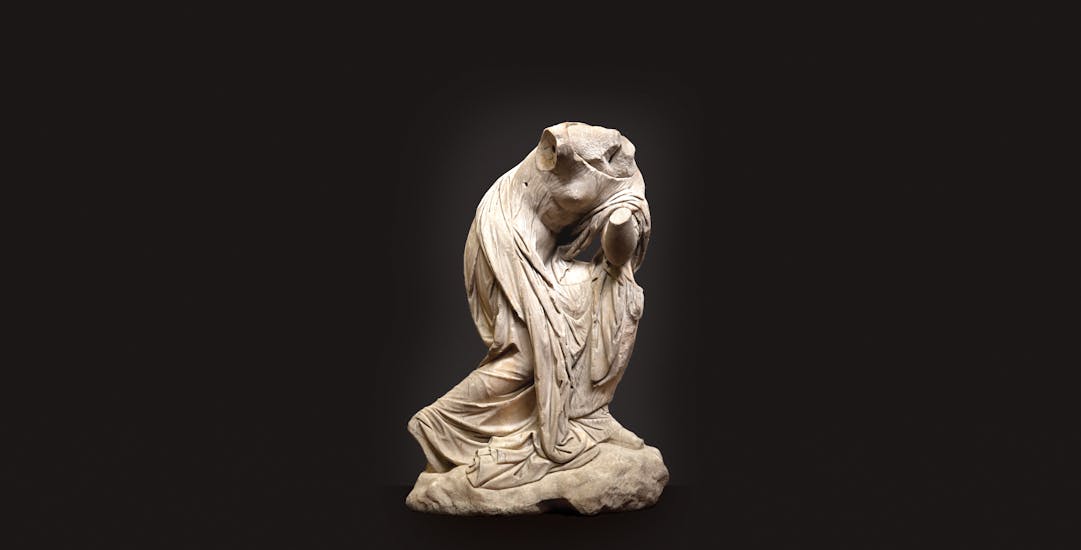This landscape-orientated color photograph features a light brown marble statue of a headless, armless woman draped in a flowing robe or toga. The statue stands against a dark gray to black background with a light gray hue surrounding it. The figure, leaning to the right, is missing its right arm entirely and half of its left arm, with the remaining forearm facing upwards and draped in cloth. The intricate carving reveals the contour of the back and calf beneath the stone drapery. At the very base of the sculpture is a rock-like, cloud-shaped platform where the statue delicately places its foot. The composition highlights the delicate details of the draped clothing and the graceful yet fragmented stance of the ancient-looking figure.